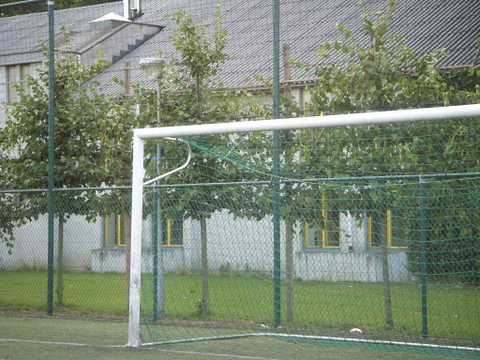This detailed photograph captures an outdoor scene focused primarily on a soccer goal. The soccer goal itself dominates much of the image, with its white frame outlining the top and sides, and a green netting that wraps around the back. The goal is positioned on a marked soccer field, evidenced by the visible baseline that runs straight through the middle of the goal area.

Behind the soccer goal stands a tall, green chain link fence, adding a layered depth to the composition. Beyond the fence, there's a row of leafy, green trees whose branches begin midway up their trunks and extend upwards. These trees provide a natural backdrop and are filled with dense foliage.

In the farthest depth of field, a large white building stretches across the length of the image. This structure features a triangular, shingled roof and numerous windows with yellow frames, contributing to its somewhat aged and worn appearance. The entire scene is devoid of people, creating a serene, almost static atmosphere. Bits of paper scattered on the ground add a touch of realism, suggesting recent human activity. 

Together, the soccer goal, fence, trees, and building create a layered and richly detailed visual narrative.